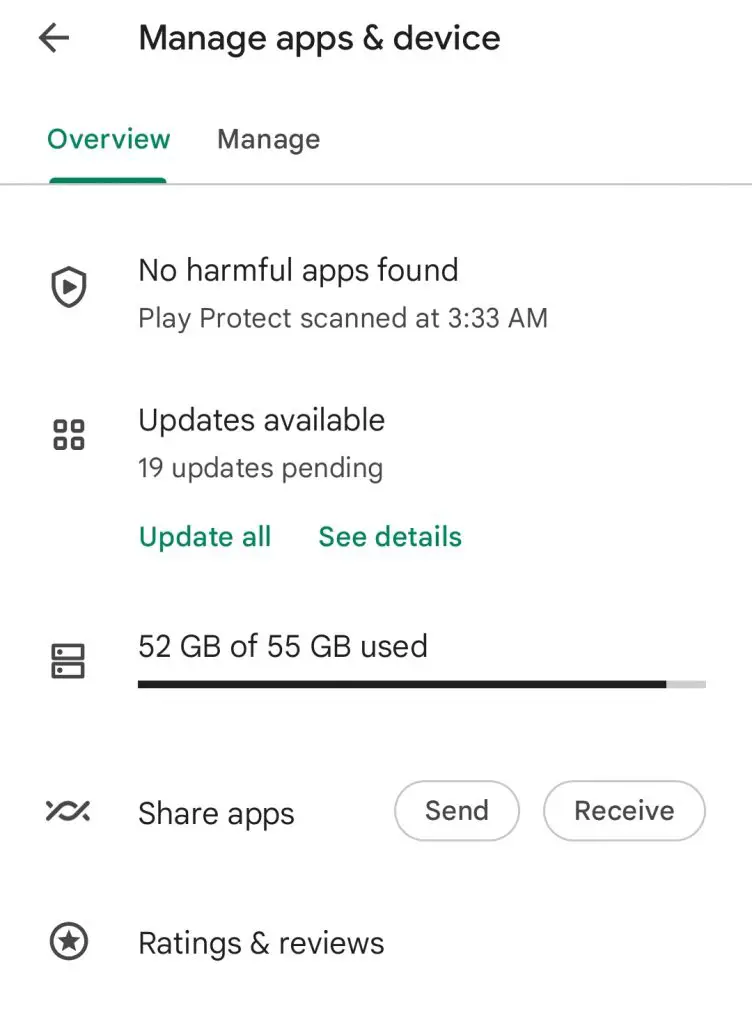This detailed caption describes the visual elements found on the "Manage Apps and Devices" screen of a mobile phone, specifically highlighting the interface for app protection and updates:

---

The "Manage Apps and Devices" screen on this mobile phone showcases several features aimed at ensuring device security and managing app updates. At the top, a left-pointing arrow is displayed next to the title "Manage Apps and Devices" in bold black text. Directly below, there are two menu items: "Overview" and "Manage". The "Overview" menu is highlighted in green with a line underneath it, indicating it is the currently selected tab.

A light gray separator line follows, beneath which a shield icon with a Play button inside signifies the Play Protect feature. The status message reads "No Harmful Apps Found," followed by the text "Play Protect scanned at 3:33 AM," reassuring the user of recent malware scans.

Below this status message, four squares are displayed next to the text "Updates available: 19 updates pending." Two green links labeled "Update All" and "See Details" provide quick access to manage these updates.

The screen also indicates storage usage with the text "52 GB of 55 GB used," accompanied by two stacked rectangles on the left. Inside these rectangles are small circles, possibly representing usage divisions, and a nearly full bar graph depicts the used storage space in black.

Further down, an icon resembling an intertwined 'V' and upside-down 'V', suggestive of a rope knot, is associated with the option to "Share Apps," featuring "Send" and "Receive" buttons.

Finally, a circle containing a star is paired with the text "Ratings and Reviews," inviting users to rate and review their apps.

---

This comprehensive caption provides a clear and detailed description of the various interface elements present on the "Manage Apps and Devices" screen.